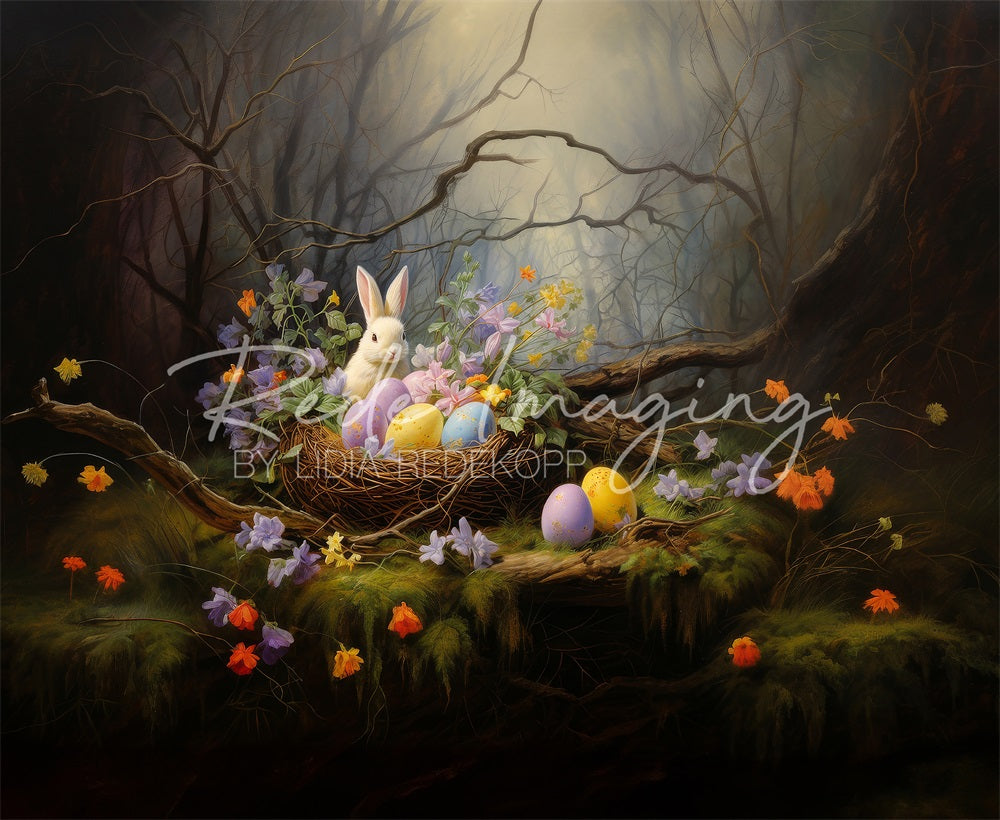This large, square, animated image features an Easter-themed scene under the title "RedE Imaging," prominently displayed in light gray, transparent handwriting across the center. Below, it credits Lydia Redekopp (spelled R-E-D-E-K-O-P-P) in all caps white text. 

The backdrop is a moody, dark forest with a gradient sky that fades from deep black in the upper left corner to a subdued brown and gray cloudy expanse in the upper middle. Here, bare, barren tree branches frame the scene, creating a canopy around this tranquil woodland setting. 

Central to the image is a charming, animated white bunny facing the viewer. It sits expectantly before a nest-like basket brimming with pastel-colored eggs, including speckled varieties in yellow, blue, and several shades of purple. In front of the bunny, on a patch of grass that seems slightly mossy and laden with atmosphere, lies a purple egg and a pink egg.

Surrounding the nest and scattered across the grassy floor are vibrant flower petals in hues of yellow, orange, and purple, adding to the whimsical and colorful Easter motif of this enchanting digital artwork.